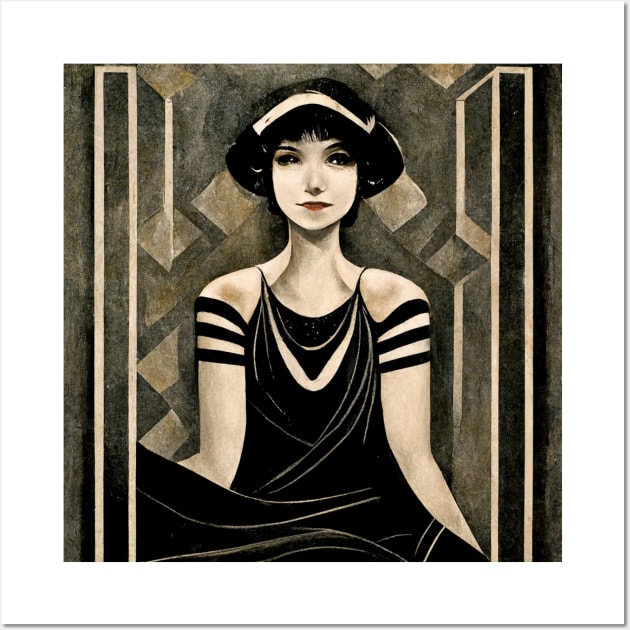This is a carefully detailed painting of a light-skinned woman with short black hair styled up, adorned with an apricot-colored headpiece. She has a striking appearance with dark eyes, bold red lipstick, and black eyeliner. She wears a black, elegant dress with spaghetti straps and additional decorative straps hanging from just below her shoulders. The dress is flowy and reaches down to about her hips, with the top part of her legs visible. The woman sits in a central position, framed by a white border.

The background is heavily textured, featuring muted and neutral tones of black, tan, beige, and hints of an apricot color, with a pattern of sponge-painted squares. It appears to resemble a decorative stone wall, contributing to the overall sophisticated yet slightly nostalgic atmosphere of the image, reminiscent of early 20th-century portraiture. The mixture of colors in the painting includes whites, grays, browns, mustard orange, and some muted reds, with no text present in the image. The woman’s expression is somewhat ambiguous, giving the impression of a subtle smirk, enhancing the painting's intriguing and classic vibe.